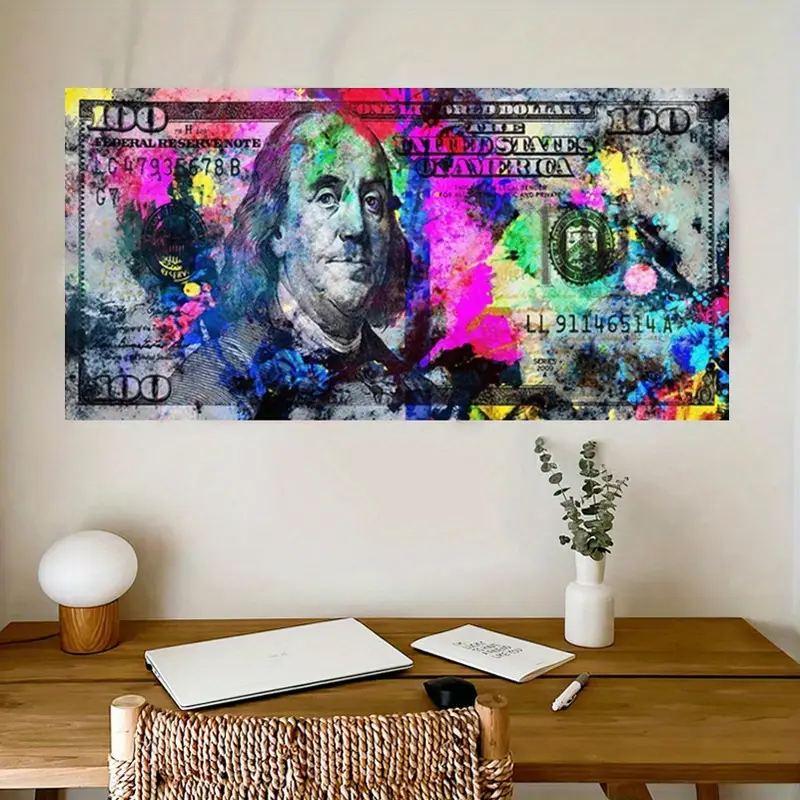The image features a chic office setup with a prominent brown wooden desk and matching chair, which has a woven backrest. On the desk lies a white portfolio, a pen or marker, a brown notebook, a laptop, and a computer mouse. A white vase with green foliage adds a touch of freshness to the space, accompanied by a unique wooden lamp with a large round bulb on a wooden cylindrical base. The backdrop is a white or light gray wall embellished with a striking, colorful depiction of a US $100 bill featuring Benjamin Franklin. This artwork covers most of the wall and is vividly painted with splashes of pink, blue, yellow, green, purple, and occasional black and tan edges, lending an avant-garde aesthetic to the room.